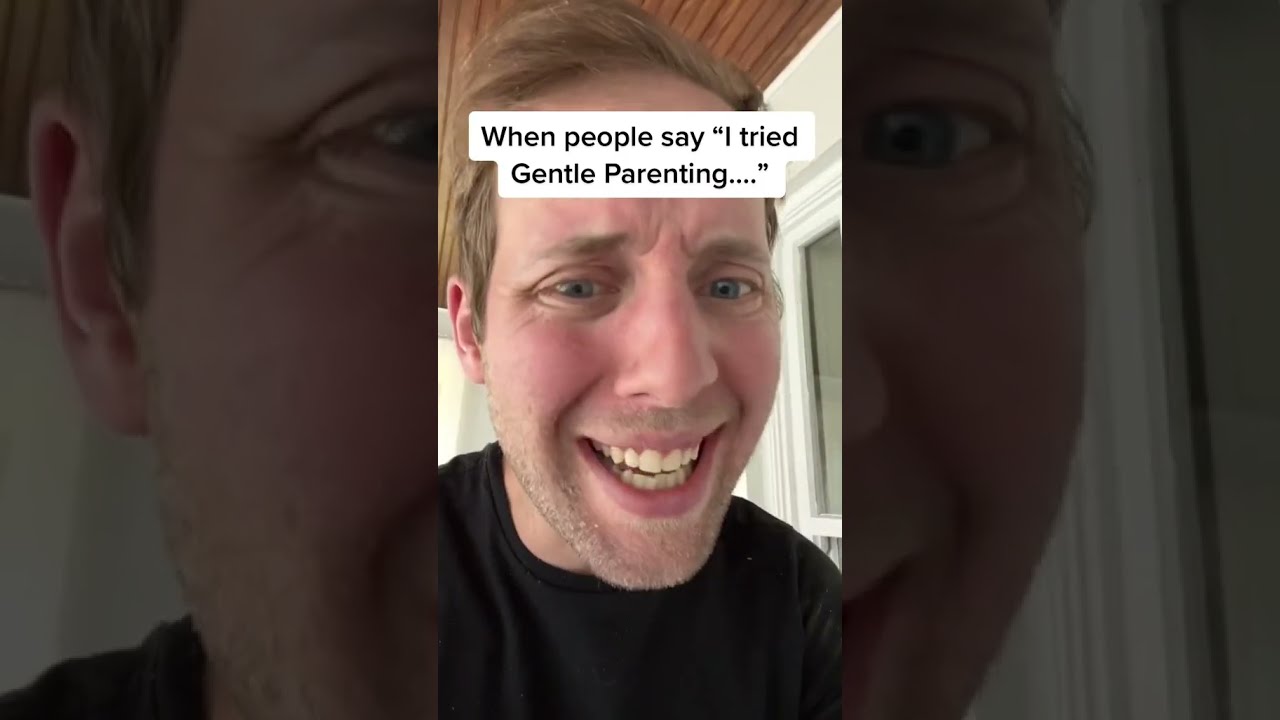The image portrays a close-up of a white man looking at the camera with an incredulous expression, as if questioning, "Are you serious?" His lips are slightly parted, revealing white teeth, and his eyebrows are scrunched together. He has blue eyes, a five o'clock shadow, and short, brownish-blonde hair with a receding hairline. His cheeks are slightly reddish. The man is framed against a background that includes a brown wooden slatted roof and a white window on his left, suggesting he's indoors, possibly in a room with white walls. Superimposed on the image is a chat bubble with black letters that reads, "When people say I tried gentle parenting..." The same picture of the man's face is faintly mirrored in the background, adding a layered effect to the composition. He is wearing a black t-shirt, emphasizing his casual attire.